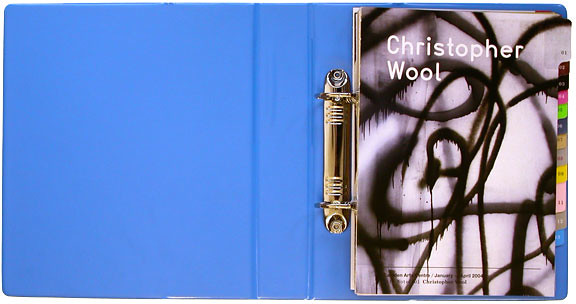The image showcases a close-up view of a planner or binder. The binder itself, seen on the left, has a brass-colored binding with a distinct, thick, finger-like protrusion and two rings. The majority of the image background is a light pastel blue. The planner's front cover prominently displays the name "Christopher Wool" printed in white lettering on a gray background, which is overlaid with black graffiti-like swoops and loops. Down the right side of the planner are multiple tabs colored in sequence from top to bottom: gray, burgundy, dark blue, pink, lime green, blue, tan, light pink, taupe, and bright blue. The planner is positioned more toward the right side of the image, showcasing the detailed, multicolored tabs that help organize the contents within.